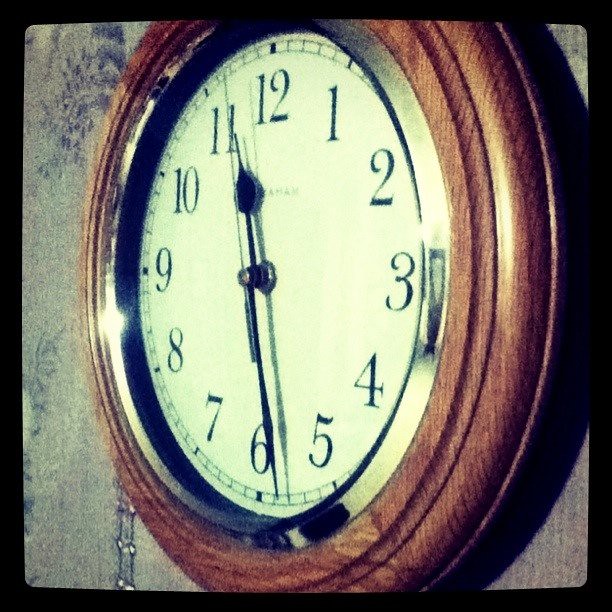A vintage-themed photograph, either authentically old or edited with a filter to appear aged, features a prominently centered clock against an indistinguishable background. The grainy, slightly blurred image adds to the antique aesthetic. The clock, with a dark wood round frame, stands out with its white face displaying black numerals. It boasts a set of black hands: a short hour hand, a longer minute hand, and a thin second hand. Despite its modern appearance, the design and presentation suggest it might be an old clock. The background remains ambiguous, potentially a gray wood grain or wallpaper, and the photo is taken at a subtle angle, making the right side slightly closer to the viewer than the left.